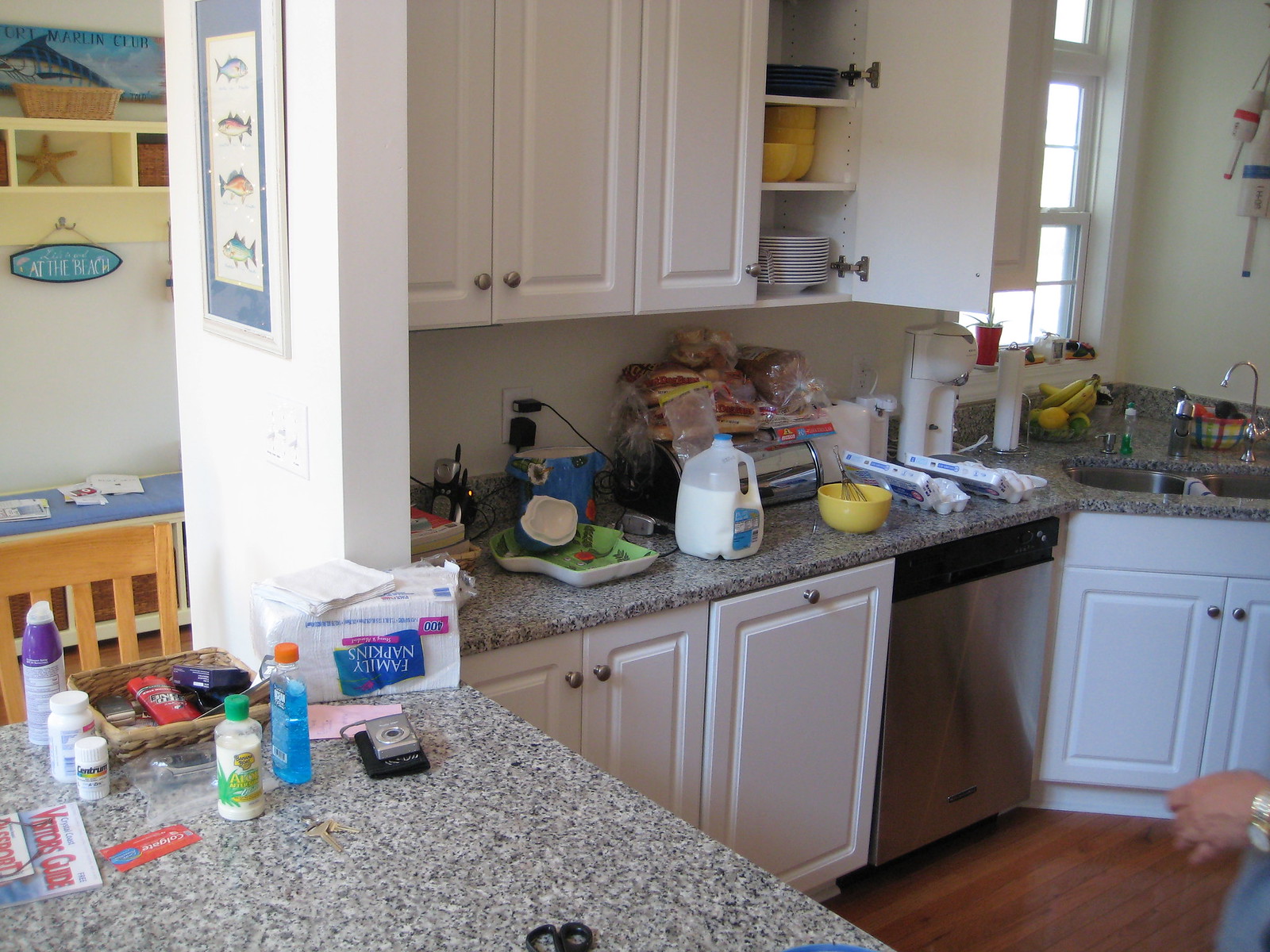This photograph showcases a well-lit kitchen with various details captured throughout the space. In the center of the image, a section of granite-like, black-and-white speckled countertops is adorned with an assortment of grocery items. Prominently featured is a jug of milk, two-thirds full, sporting a blue label. Beside it, several packages of bread rest atop a stylish black and silver bread box. The countertops are flanked by cabinets above and storage areas below.

To the right, the countertop angles off at a 45-degree turn, ending near a white wall that creates a corner in the room. In this corner, you find a kitchen sink situated below a window that allows natural light to flow in. Adjacent to the sink and slightly to the right of the main counter space is a dishwasher. 

In the bottom left corner of the image, a separate countertop holds a collection of multivitamins and a basket brimming with miscellaneous items, hinting at the coziness and lived-in nature of the space. A wooden chair is pulled up against this section of the counter, partially visible with its back facing the camera.

The bottom right corner reveals a glimpse of the kitchen's burgundy-colored wood flooring, adding warmth to the room’s predominantly white decor. Additionally, part of a person’s body is visible, with a hand reaching into the frame, contributing a candid touch to the scene. This detailed and inviting kitchen setting is captured in clear lighting, highlighting each aspect of the space.